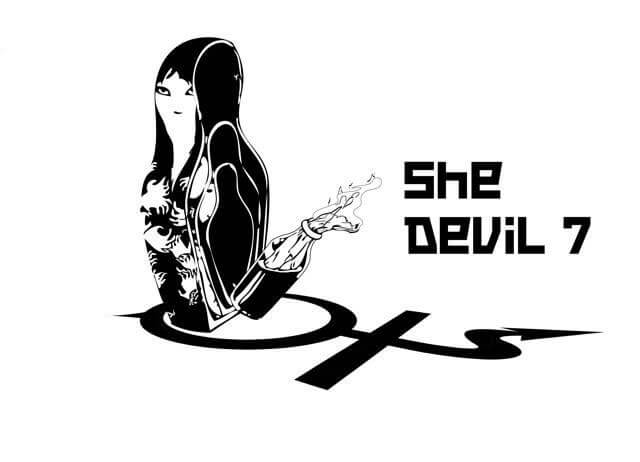This detailed black and white sketch features a striking and symbolic representation of a woman combined with elements reminiscent of a Russian nesting doll, set against a solid white background. In the left part of the image, we see the upper half of a woman, who appears to be of Asian descent, characterized by slanted eyes and long, wavy black hair that cascades down to her waist. Her image is portrayed in a series of nested layers, like a matryoshka doll, with each successive smaller version of herself revealed inside the cutaway of the larger form. At the core of these layers, instead of another doll, sits a Molotov cocktail—a jar containing a black liquid with flames erupting from its top. This smaller, fiery bottle stands centrally on a black circle which may symbolize a female gender symbol, but with a twist: the circle's tail extends outward like a devil's tail.

The image balances on this symbolic figure with additional distinctive elements: the woman's image appears to rest on or is integrated into the black circle, combining to create a half-body shape atop this platform. The right side of the composition is dominated by bold black capital letters that spell out "She Devil's Seven" or "SheDevils7," adding a strong textual element that suggests a thematic or titular significance, such as a title for a game or a movie. The overall effect is a multifaceted piece brimming with dark, metaphorical undertones.